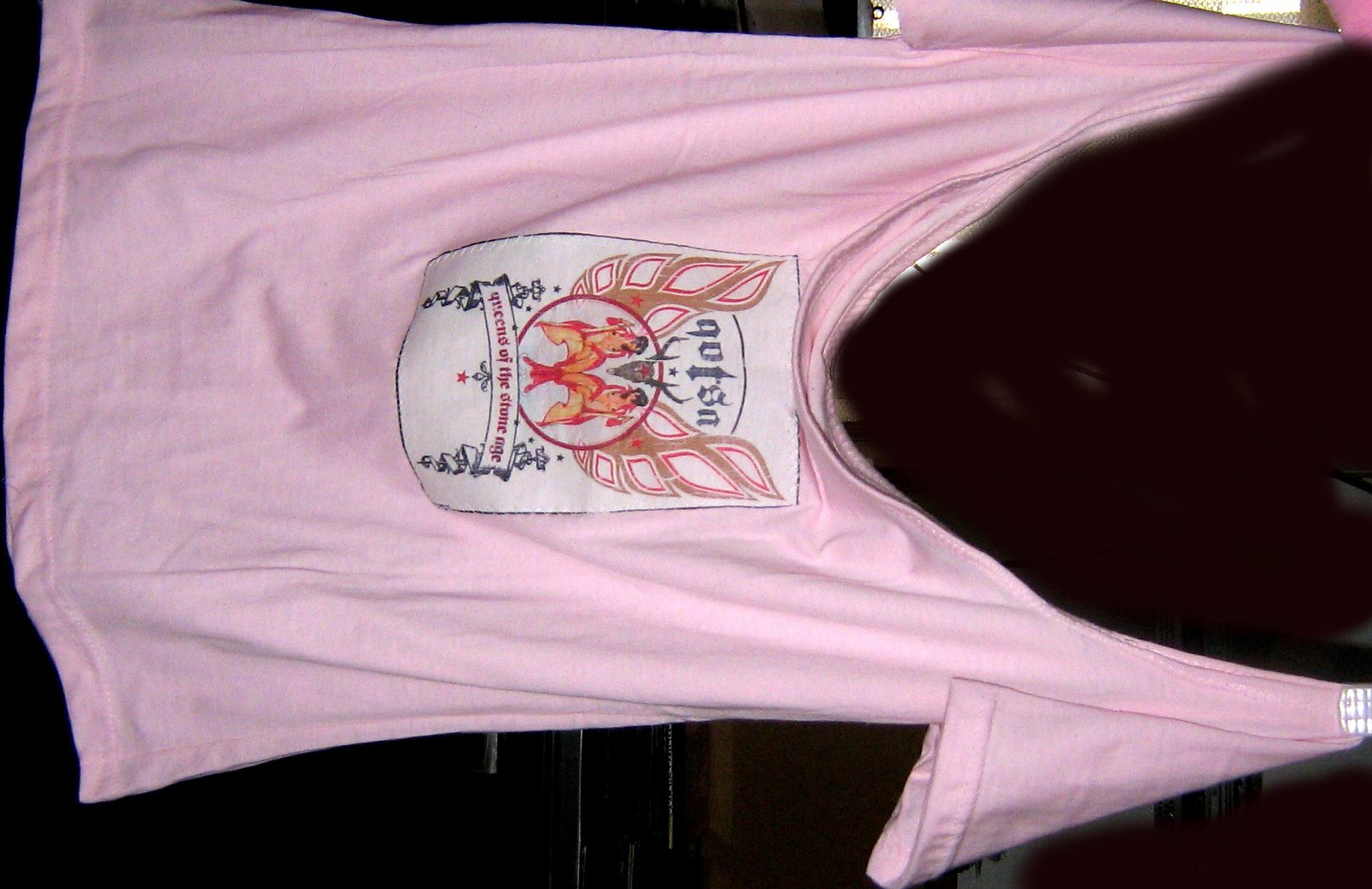The image shows a pink shirt hanging sideways, seemingly on a wall inside a house. The orientation of the photo makes it a bit challenging to discern the precise context. The shirt is entirely pink and appears to have had something near the collar area that has been either photoshopped out or painted over with black, possibly using a simple tool like MS Paint.

On the mid-right side of the shirt, there is a detailed logo. This logo features pairs of wings, gold in color with white and red trim on the inside, arranged symmetrically. Between the wings, two female figures are depicted sitting in a circle with what appear to be towels around them and pasties covering their breasts. Above them is the image of a deer head with antlers.

The text on the shirt reads "Q-O-T-S-N," which seems to stand for "Queens of the Stone Age," indicating that this might be a band T-shirt.